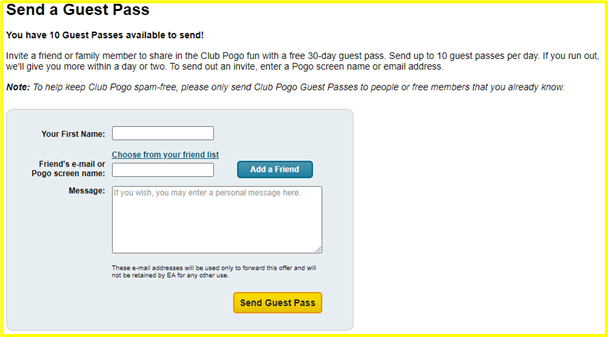The image features a detailed promotional section from a website, adorned with a thin yellow border. Set against a white background, the top left corner prominently displays the phrase "Send a Guest Pass" in bold black letters. Just below, in similarly bold black text, the message reads, "We have 10 guest passes available to send!" followed by an exclamation mark.

A subsequent space is followed by an informative paragraph, explaining, "Invite a friend or family member to share in the Club Pogo Fun with a free 30-day guest pass. Send up to 10 guest passes per day. If you run out, we'll give you more within a day or two. To send out an invite, enter a Pogo screen name or email address."

Beneath this text block is a cautionary note emphasizing, "To help keep Club Pogo spam free, please only send Club Pogo guest passes to people or free members that you already know." 

To the right of these instructions, a section against a light blue background provides fields for inputting your first name, a friend’s email or Pogo screen name, and a message. At the bottom of this section is a yellow box with the directive, "Send Guest Pass."

The bottom right of the image is simply blank white, creating a clean and uncluttered look.